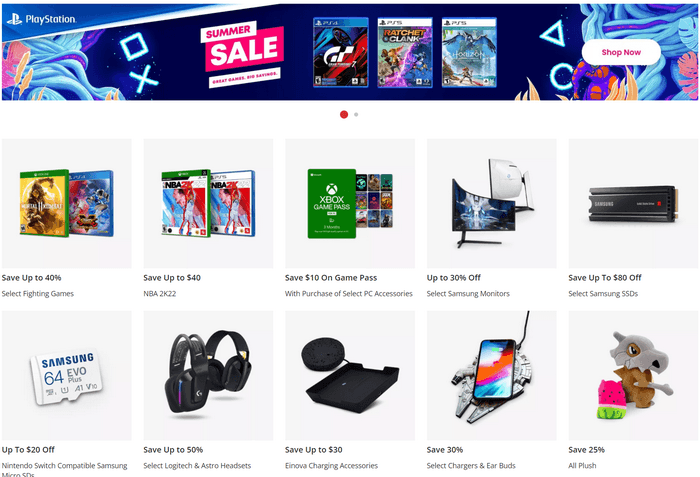This image is a cropped screenshot of an electronic store's desktop website with a predominantly white background. At the top of the page, there is a large banner dedicated to PlayStation, featuring the PlayStation logo in the top left corner. In the center-left area of the banner, bold text announces a "Summer Sale," while to the right, there are three thumbnail images of PlayStation video game covers. Further right, a prominent white button labeled "Shop Now" invites users to make a purchase.

Beneath the banner, the background remains white, and two small dots appear at the center, likely indicating pagination. The first dot is bright red, suggesting that this banner is the first of two images or that this page is the first of two sections.

Following the banner, the main content displays two rows of product thumbnails, each row containing five items. In the first row, the products and their promotions are as follows:

1. Two video games with a caption stating "Save Up to 40% on Select Fighting Games."
2. Adjacent to it, an offer that says "Save Up to $40 on NBA 2K22."
3. In the center, a box showcasing the Xbox Game Pass, accompanied by the message "Save Dollars on Game Pass."
4. Next, two images of a curved gaming monitor with the label "Up to 30% Off Select Samsung Monitors."
5. The last item in the first row promotes Samsung SSD Cards with a deal stating "Save Up to $80 on Select Samsung SSD Cards."